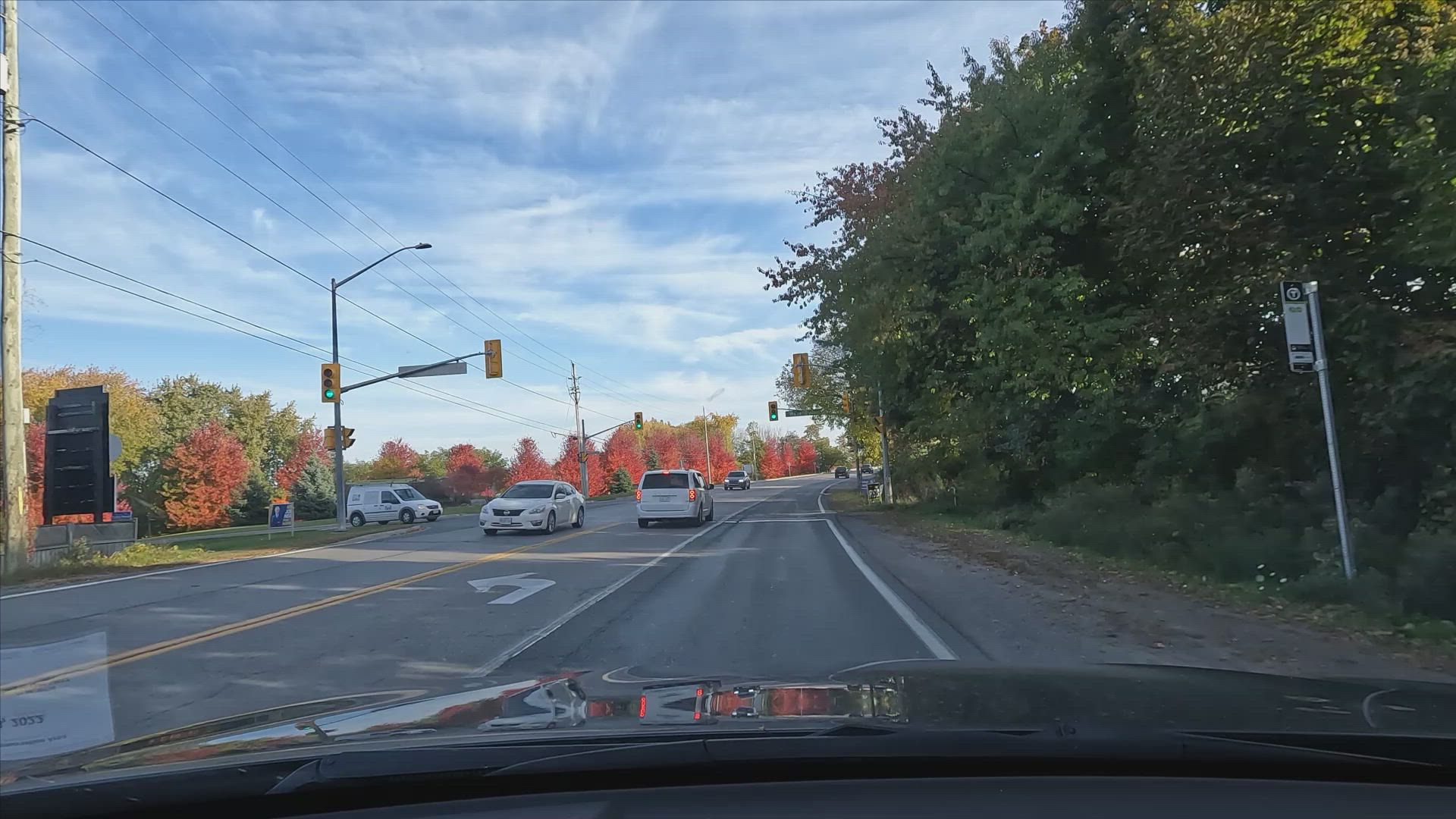This is a rectangular dashcam image taken from the inside of a vehicle positioned in the far right lane of an asphalt street at an intersection. The long side of the rectangle spans from left to right. The interior of the vehicle reveals the hood and the end of the dashboard, along with a windshield wiper in its resting position. The vehicle has the green light to proceed forward.

Outside, the scene is lively with traffic and urban elements. To the left, there is a turn lane with a white van preparing to make a turn, while another vehicle travels in the opposite direction. Ahead, a white van is positioned in the straight-through lane, facing away from the camera. Another vehicle, a white car, is about to turn right into the opposing lane from the intersection. The road is marked with white directional arrows and yellow double lines in the center.

On the right side of the image, there is a street sign, possibly indicating a bus stop, and streetlights illuminating the way. Dense shrubbery and deciduous trees, some with leaves turning red, border the road, hinting at the fall season. Above, the sky is a mix of bright blue hues with smeared, scattered clouds, creating a hazy atmosphere.